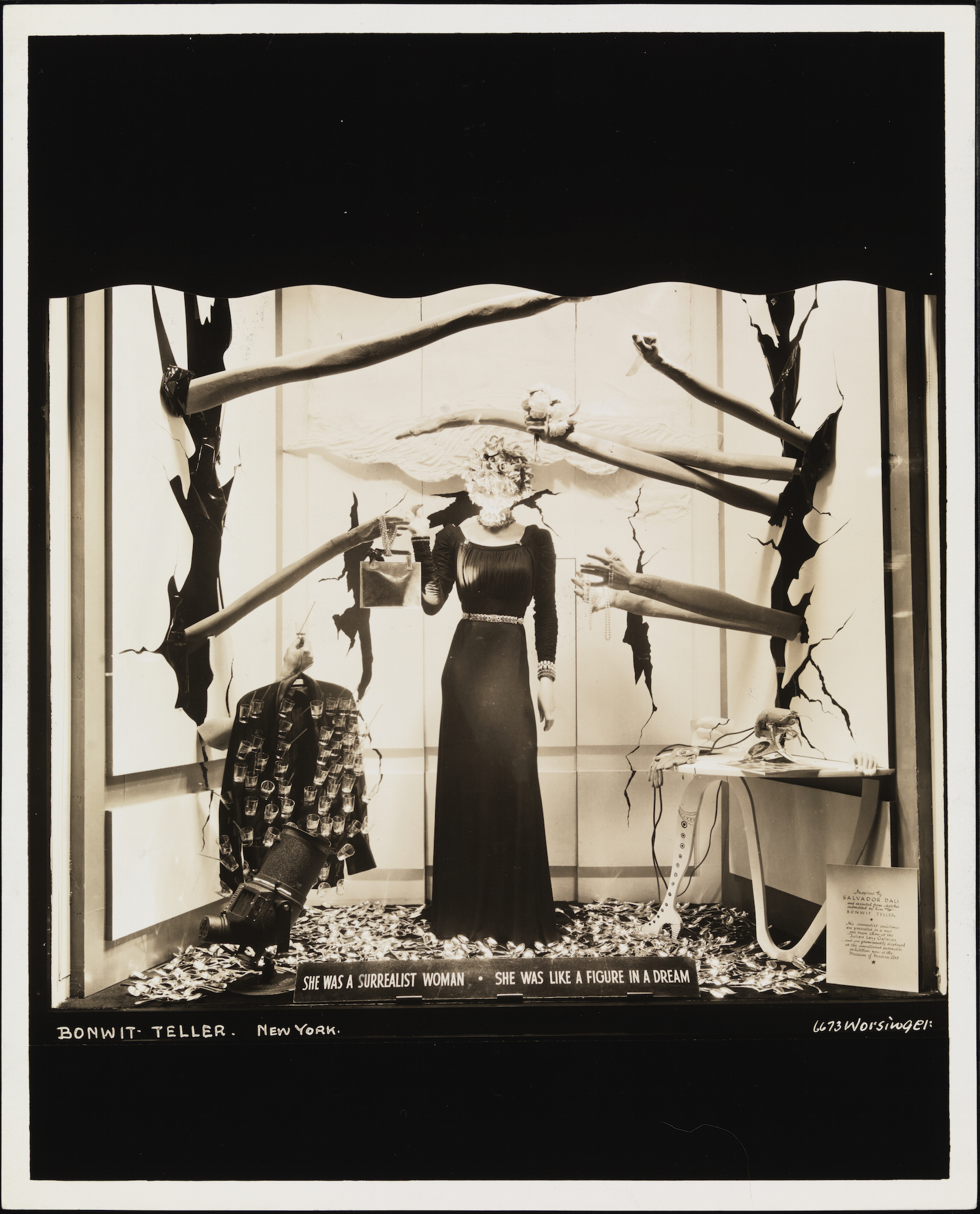The image features an evocative, surreal scene rendered in a limited palette of black, white, and sepia tones. The composition is framed by a black area at the top and bottom, and enclosed within a white border. At the center stands an enigmatic female figure, her face obscured or blurred, adorned in a long-sleeved, dark-colored gown that cascades to the floor and cinches at the waist with a belt. The walls surrounding her are cracked and give the illusion of hands reaching out toward her from all directions, intensifying the surreal atmosphere. 

To the left of the scene, a black jacket is visible, and to the right, there appears to be a table or desk. The entire illustration is highlighted by a light that casts a focus on the mysterious woman, enhancing her dreamlike presence. Below the image, text reads: "She was a surrealist woman, she was like a figure in a dream," followed by "Bonwit Teller, New York." Additional text to the right mentions "6673 Worsling, EL." The overall visual effect combines elements of art and fashion into a hauntingly surreal tableau.